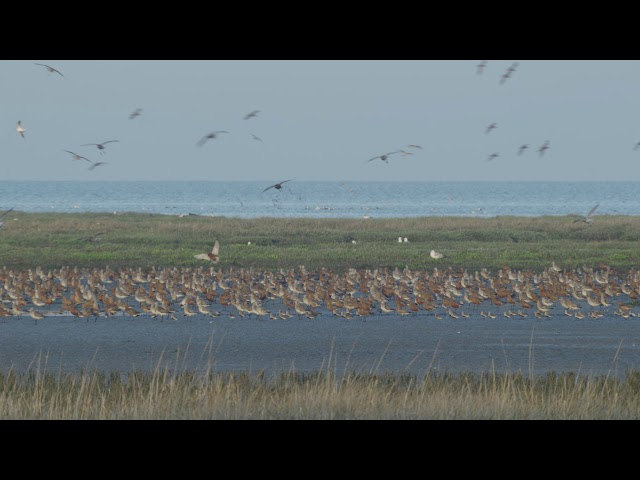In this low-quality landscape photograph, we observe an outdoor scene teeming with seabirds, likely seagulls, situated near a vast body of water, probably the ocean or a large lake. The foreground features stretches of dry, tall grass, transitioning into a marshy area where a pond or stream is brimming with brown and white birds. Some birds are also captured in flight, albeit blurry due to the movement and the image's low resolution. Beyond the marshland fragments, another expanse of grass leads up to the larger ocean or lake, visible on the horizon. The sky above is a murky grayish-blue, creating a somber backdrop for the bustling activity below. The photograph is framed by black bars at the top and bottom, reminiscent of a widescreen movie format.